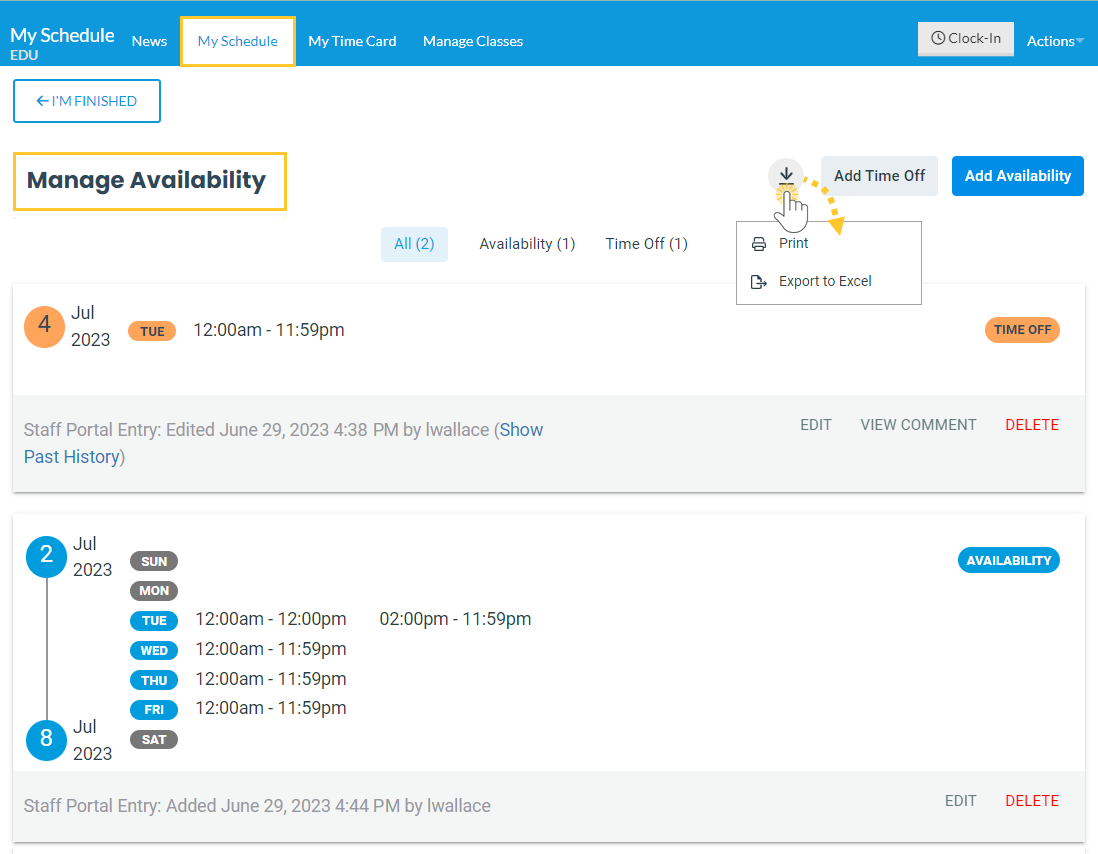A screen capture from an educational application is displayed, specifically showing the "Manage Availability" section within the "Staff Portal Entry" as of July 4th, 2023. The app includes various features accessed via tabs labeled "News," "My Schedule," "My Timecard," "Manage Classes," and "Clock In." There's also a navigation button labeled "I'm Finished" with an arrow, indicating a return to the previous screen.

In the "Availability" section, the system provides schedule details for the week of July 2nd through July 8th. According to this schedule, staff are available on Tuesdays, Wednesdays, Thursdays, and Fridays. However, availability is marked as unavailable on Sunday, Monday, and Saturday.